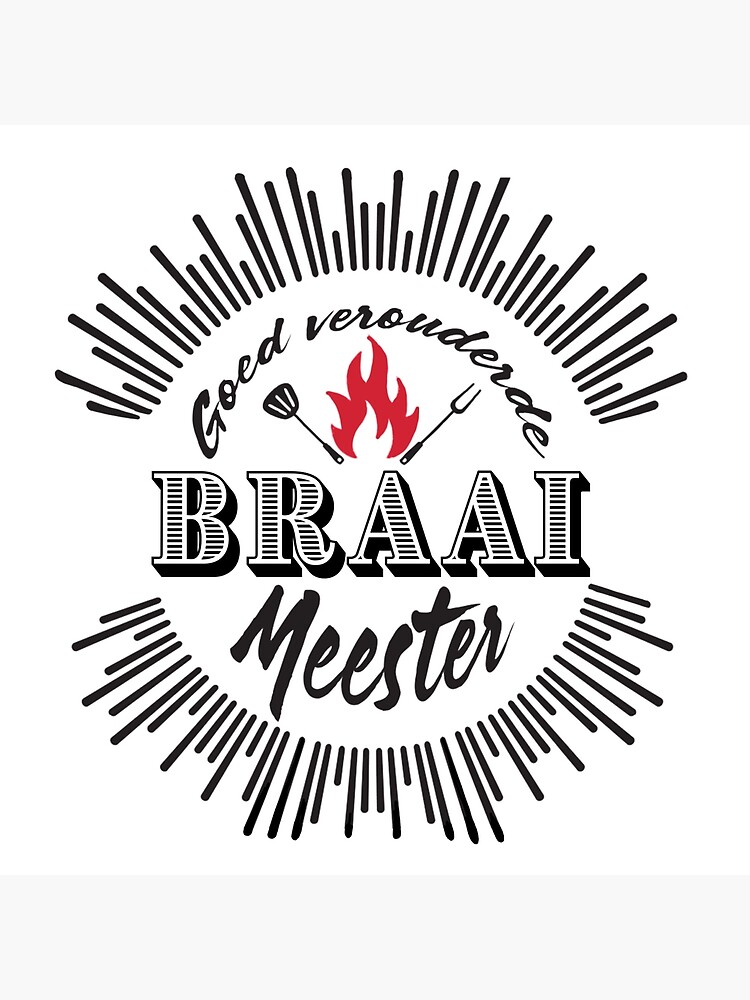The image showcases an advertising label featuring a central white background with the text "GOED, V-E-R-O-U-D-E-R-A-D-E." Surrounding the text are black lines radiating in a semi-circular pattern from both the top and bottom, creating a striking visual effect. In the center, there is a red flame flanked by a spatula on the left and a fork on the right. Beneath this, the word "BRAAI" appears in bold black and white letters, followed by "MEESTER" written below. The overall design resembles a label typically found on a bottle, with a dynamic blend of black and white typography accented by the red flame.